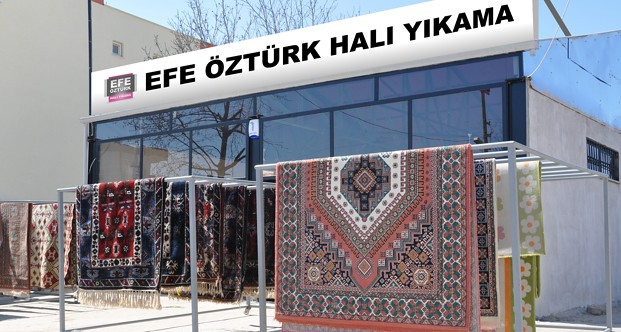The image depicts an outdoor scene featuring a rug store specialized in displaying and selling various area rugs. In the background, a clear blue sky is visible along with tree branches extending beyond the shops. The setting includes a large white building to the left, next to which stands a tall tree. In the foreground of the photo is a smaller white building with a full glass storefront, topped by a white sign with black lettering that reads "Efe Ozturk Hali Yakama," set within stylized rectangles.

In front of the store, three sturdy metal racks are embedded in the concrete ground, each draped with an assortment of area rugs. These rugs, predominantly featuring intricate oriental patterns, exhibit a range of colors including shades of navy blue, red, green, and white. Among the collection are some rugs with more Western designs; for example, one rug has a grass-green background adorned with stylized daisies. Noteworthy are an orange and brown rug with an orange border, another with burgundy and blue tones, and a dark black rug. Each rug, with its unique pattern and color scheme, adds to an overall vibrant display that catches the eye of passersby.